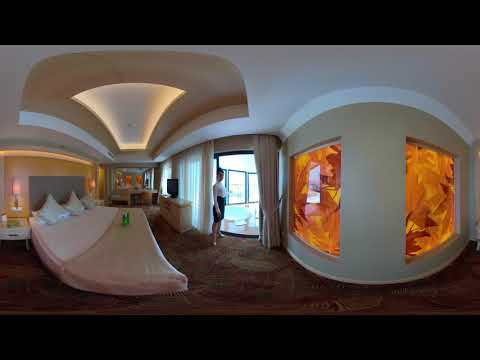The image depicts the interior of a spacious, tastefully decorated room, possibly a hotel suite or a modern apartment. The focal point is a large, wide bed on the left side with three pillows and a light tan covering partially masking its base. A green box rests atop the bed, which is flanked by two compact, orange-hued bedside tables, each topped with a small table light. The wall behind the bed is a dark yellow shade, while the floor is a reddish-brown color.

In the center of the room, a woman stands near a well-lit sliding door or large window. She is dressed in a white long-sleeved shirt and a knee-length black skirt with high heels. Her hair is styled in a bun. Beyond the door, there's a glimpse of a sophisticated outdoor area, featuring what appears to be a small pool or jacuzzi, framed by additional square windows.

To the right, a curved wall showcases two large orange decorative pieces that resemble oversized fall leaves embedded in glass panes. The right side also features a TV and a dresser. There is a wide table in the background with two chairs pushed against it, a mirror reflecting the room's opposite side, and the ceiling displays a unique fan-shaped inset with built-in lighting.

Overall, the room blends warm tones of white, yellow, beige, and orange, creating a cozy yet elegant atmosphere, enhanced by carefully selected furniture and decoration.